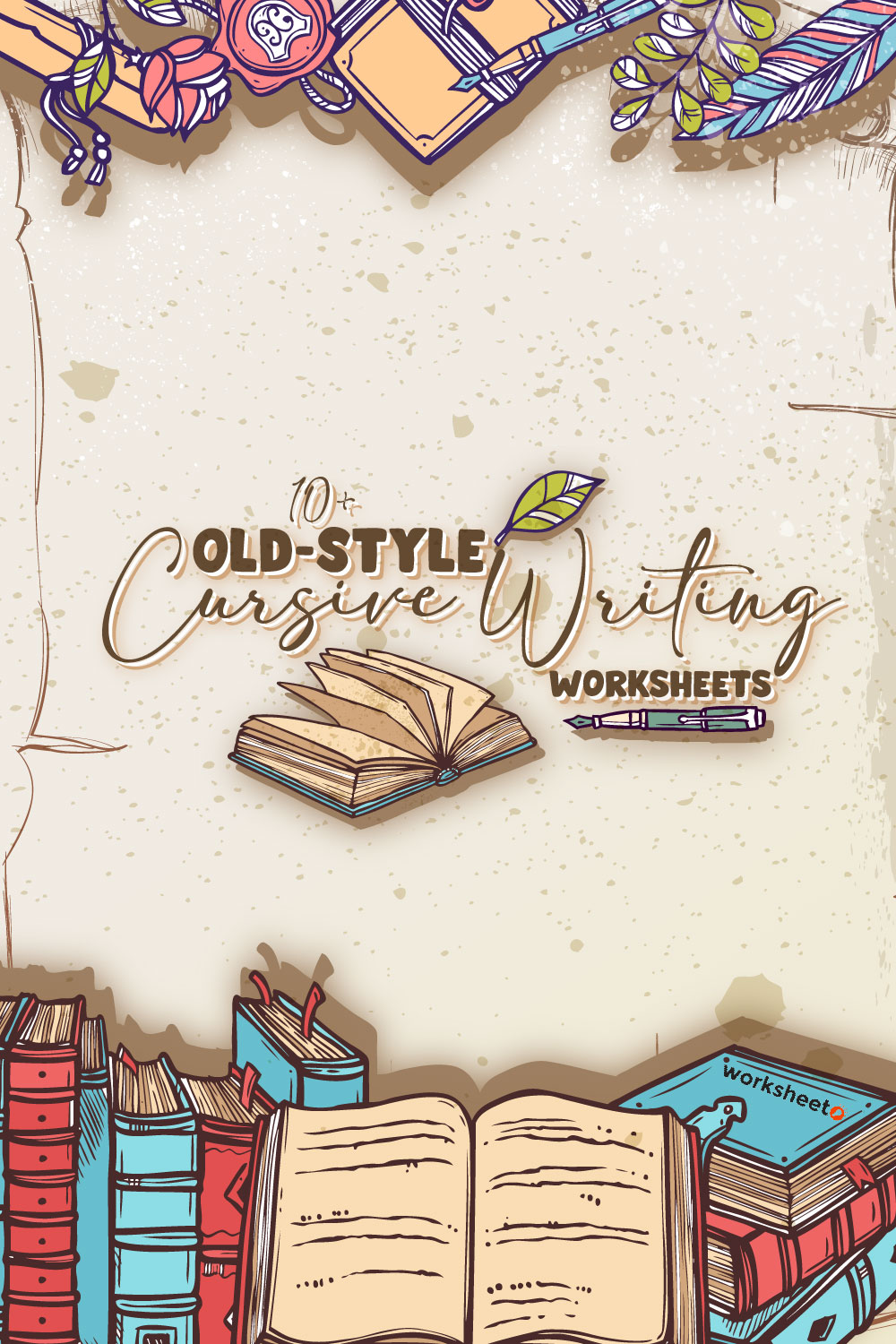This image appears to be a hand-drawn poster or book cover primarily designed to promote "10+ Old-Style Cursive Writing Worksheets." The background of the poster is tan with darker tan specks, giving it a vintage feel. 

In the middle of the poster, the title "10+ Old-Style Cursive Writing Worksheets" is prominently displayed in a combination of thin black handwritten font, bold all-caps brown font with a white outline for depth, and black cursive. Beneath the word "cursive" is an open book with its pages fanned out, and underneath "worksheets" is an illustration of a fountain pen.

The bottom section features a lineup of blue and red books, each with little red markers protruding from them, adding vibrant detail to the image. At the very bottom, there's another open book.

The top part of the poster showcases an array of intricate, hand-drawn designs, including feathers, leaves, and another fountain pen, all of which contribute to the overall artistic and hand-crafted aesthetic of the poster. The exact nature of the items at the top is unclear, but the designs add to the richness and detail of the image, indicating a theme tied closely to handwriting and traditional writing implements. The viewer remains uncertain if it's an advertisement or the cover of the cursive writing worksheets themselves.